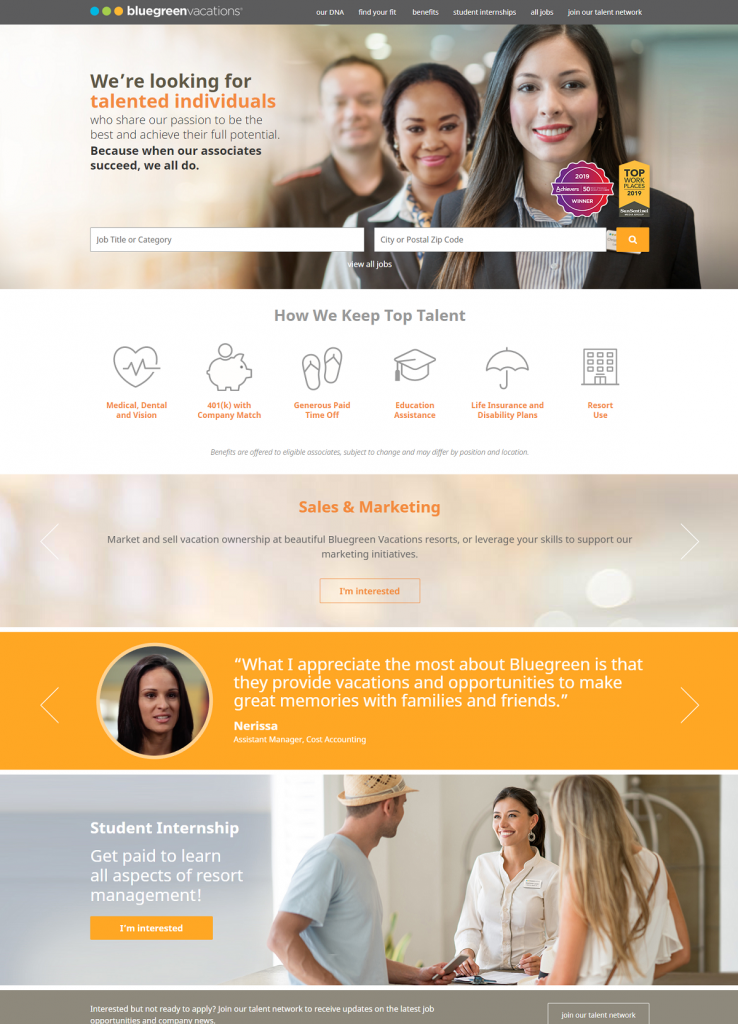Caption: 

The homepage of the Blue Green Vacations website showcases an inviting call-to-action, encouraging talented individuals to join their team and unleash their full potential, underscoring the collective success achieved through individual growth. The page, albeit generic in design, unfolds into various sections as one scrolls. Initially, a search bar for job titles and categories appears, likely part of the careers section. Further down, the segmentation seems less defined as both "Sales and Marketing" and "Student Internship" are introduced. The Sales and Marketing section focuses on marketing and selling vacation ownership, with an "Interested" button available for engagement. Below, the Student Internship segment promotes a paid learning opportunity covering all facets of resort management, highlighting the company's commitment to education and practical experience in the resort industry.